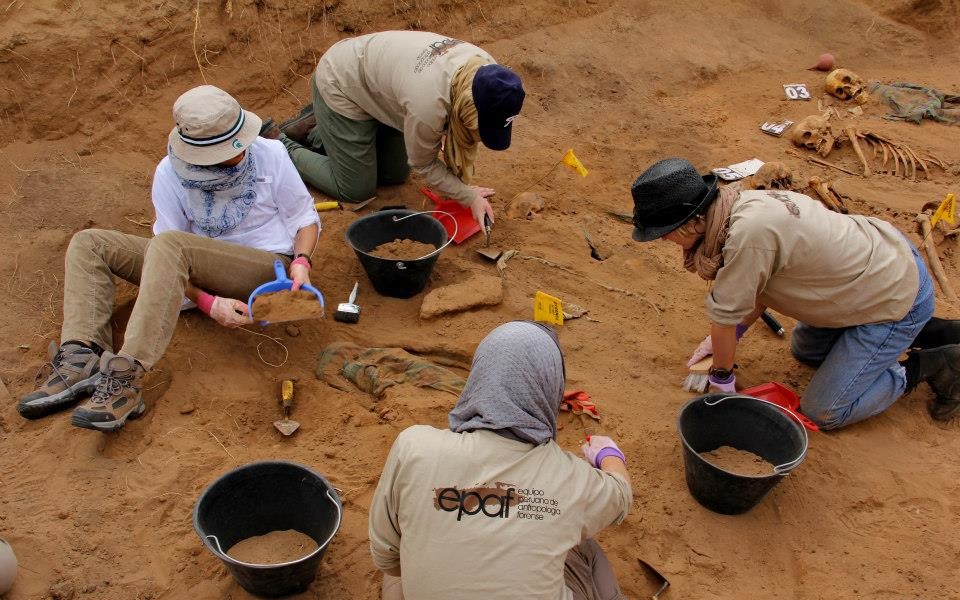This image portrays an archaeological dig site featuring four individuals diligently excavating in a sandy area. They are dressed in casual attire consisting of t-shirts, long pants, and protective headgear such as scarves, masks, and hats, indicating their preparation for the desert-like conditions. Three of them are wearing t-shirts with the acronym "EPAF" prominently displayed, alongside some indistinct text. Scattered around them are various tools including shovels, trowels, paintbrushes, and dustpans, highlighting their meticulous excavation process.

In the midst of their work, there is a piece of cloth partially buried in the sand, potentially the focus of their digging. Surrounding them are three green buckets filled with sand and dirt. Notably, to the upper right of the scene, there are three skeletons—each marked with numbers 03, 04, and 05—still partially embedded in the ground. Some of these skeletons appear to be wearing remnants of blue cloth. Nearby, a couple of small flags are staked into the ground, likely serving as markers for the dig site. The vivid detailing, including the possibility of a fifth person’s knee visible at the bottom left of the image, emphasizes the collaborative effort in unearthing and studying these ancient remains.